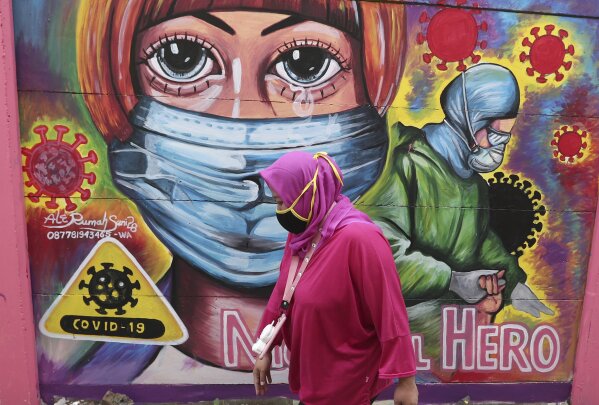In this vibrant and emotional scene, a woman dressed in a pink hoodie with the hood up and a pink lanyard with an ID around her neck walks past a striking mural. She wears a black fabric face mask with yellow trim, indicative of the COVID-19 era. The mural behind her bursts with multiple bright colors, drawing attention to its poignant message. Central to the artwork is a large, detailed face of a young girl, adorned with a COVID mask and an expressive tear in her eye, embodying the ongoing pandemic's toll. To the right of this face, a medical professional, covered head-to-toe in green personal protective equipment (PPE), including a mask, goggles, and a head covering, tenderly holds the hand of a patient, symbolizing the healthcare heroes of this crisis. Scattered across the mural are menacing representations of the COVID-19 virus, alongside a biohazard warning sign marked with "COVID-19." Partial lettering behind the woman spells out "National Hero," emphasizing the commendable efforts of frontline workers. The mural captures a powerful narrative of compassion, resilience, and the human impact of the pandemic.